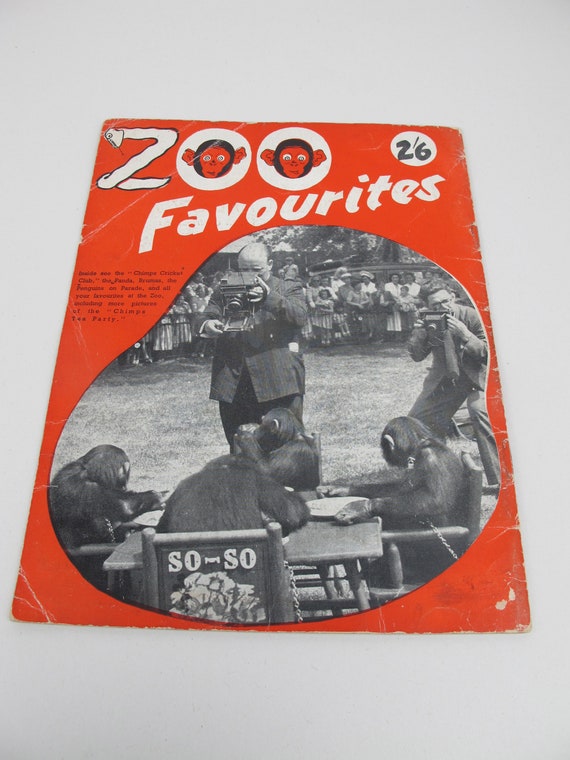This is an old, scratched poster with a primarily red background, featuring a title at the top in white letters that reads "Zoo Favorites." The double O's in "Zoo" are creatively designed with red and black drawings of monkeys, while the Z has a snake head design. At the upper right corner, there's a white circle containing the numbers "2-6" in black.

Central to the poster is a black-and-white photograph with a curved shape overlaying the red background. The photograph depicts a scene of four monkeys seated in chairs around a wooden table, eating from plates placed in front of them. Behind the monkeys stand two photographers capturing the moment, with a considerable crowd observing in the background. The poster includes some small, unreadable black text on the left side of the photograph. The entire poster, which has an off-white, grayish backdrop and some visible wear and tear, exudes a vintage charm reminiscent of bygone eras, likely highlighting a chimp's tea party event.